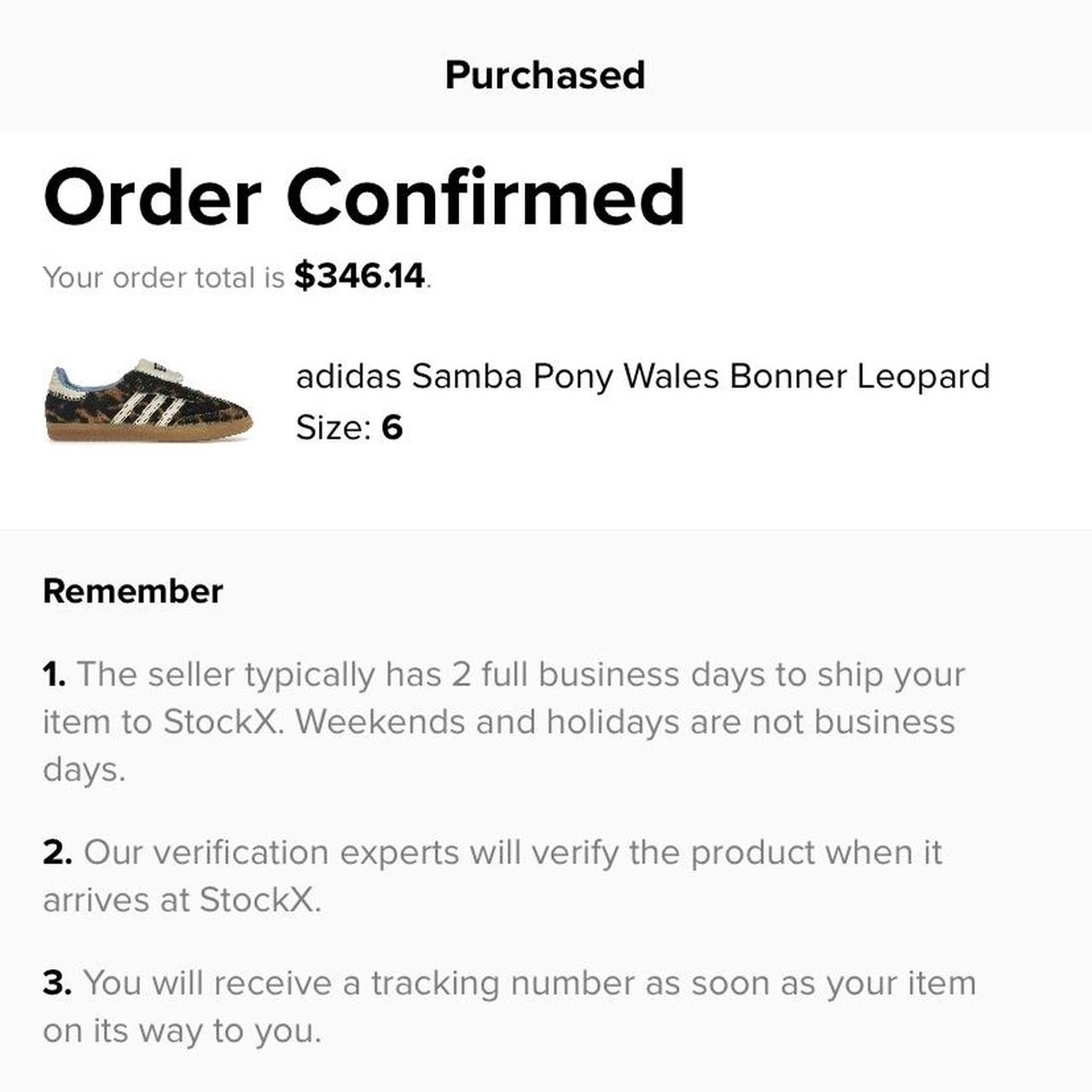**Detailed Image Caption:**

In the center of a white background is a screenshot capturing the finalization of a purchase. The word "PURCHASED" is prominently displayed in black text in the dead center. On the left-hand side, bold text reads "Order Confirmed," promising that the transaction is complete. Below this, gray text outlines the total order amount: "$346.14."

To the right, the screenshot features an image of the purchased item: a pair of Adidas sneakers with a distinctive, albeit controversial, design. These Adidas have a unique camel-like appearance with a green and tan camouflage pattern. They are accented with three white stripes on the side, a white heel, white top, and a white tongue. The model name is "Adidas Samba Wales Bonner Leopard," indicating a leopard print theme, and the sneaker size is six.

Below the product image, instructions for the post-purchase process are outlined:
1. "Remember, the seller typically has two full business days to ship your items to StockX. Weekends and holidays are not business days."
2. "Our verification experts will verify the product once it is received at StockX."
3. "You will receive a tracking number as soon as your item is on its way to you."

This screenshot encapsulates the moment someone committed to buying a pair of expensive Adidas sneakers, which they might display rather than wear, akin to paying the price of high-end electronics from years past.